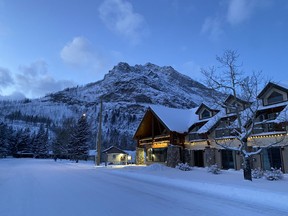In this snowy winter scene at the base of a small mountain, a large building, likely a ski lodge or possibly a hotel, stands prominently. The multi-story structure has an affluent log-cabin aesthetic, featuring multiple sections or doors, indicating it may function as a commercial establishment rather than a private home. Freshly fallen snow blankets the ground and the roof, while a recent plowing has cleared the street, leaving thicker snowbanks along the edges. The surrounding landscape includes coniferous trees and a leafless deciduous tree, all heavily dusted with snow. The backdrop reveals a towering, snow-covered mountain and an evening sky transitioning towards dusk, casting a serene bluish hue over the scene. This ambiance is softly interrupted by the warm, orange glow of lights emanating from the lodge, imparting a cozy contrast to the otherwise cool, snowy environment.